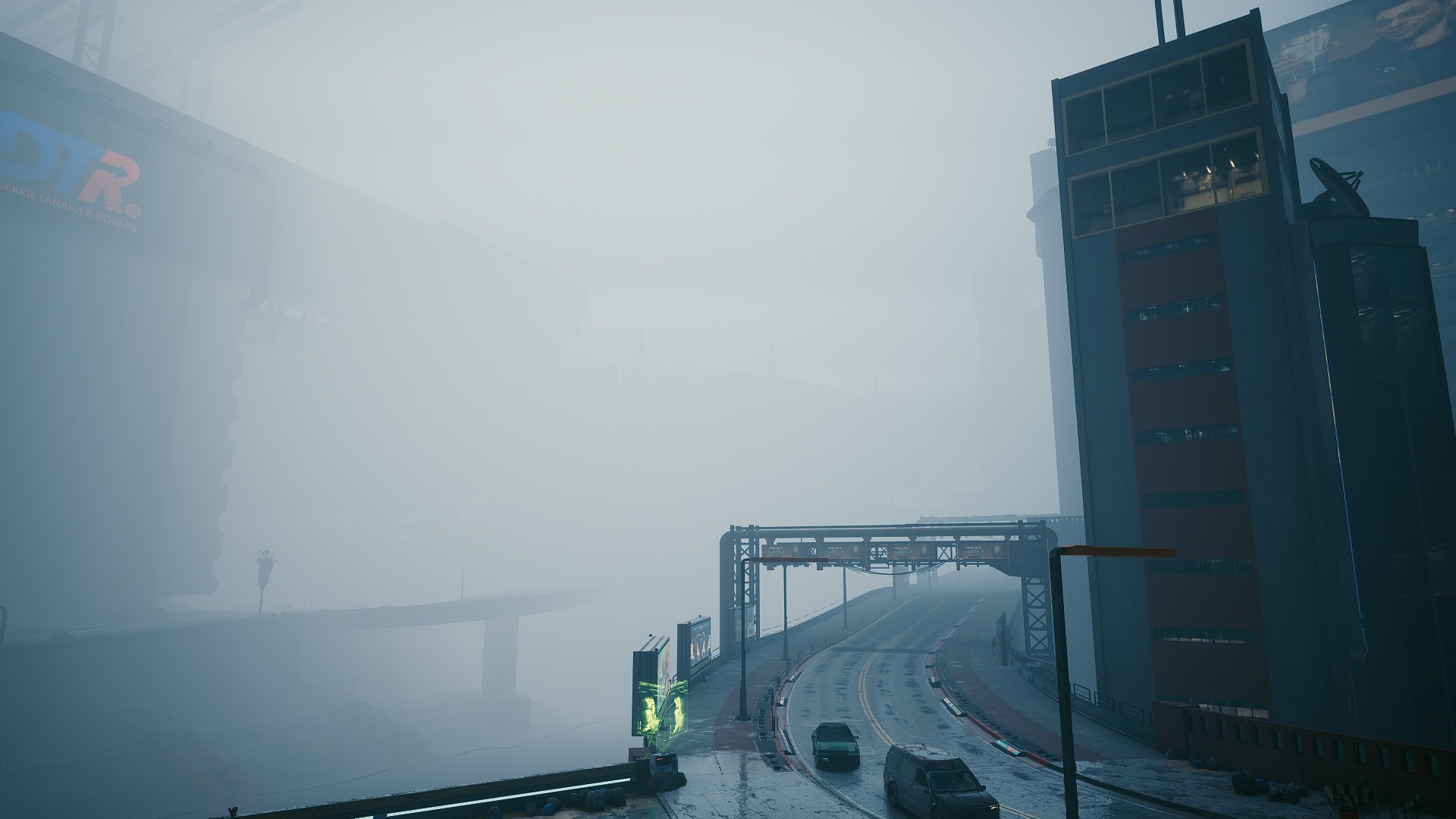This color photograph presents an ethereal urban scene where dense fog envelops the surroundings, creating an almost surreal atmosphere that blurs the line between reality and digital art. A street emerges from the obscured background, winding straight down the image before curving to the right. This road, partially hidden by the dense mist, hosts a couple of cars, their forms faint amidst the fog. On the right side, tall buildings rise, their upper stories vanishing into the haze. To the left, various structures attempt to appear through the thick fog, but their features remain largely indiscernible. The dense fog fills the space between the buildings, obscuring much of the cityscape below and adding an air of mystery to the scene. The composition focuses on the lower right portion of the frame where the street and cars are most visible, creating a moody, dreamlike vision of urban life shrouded in mist.